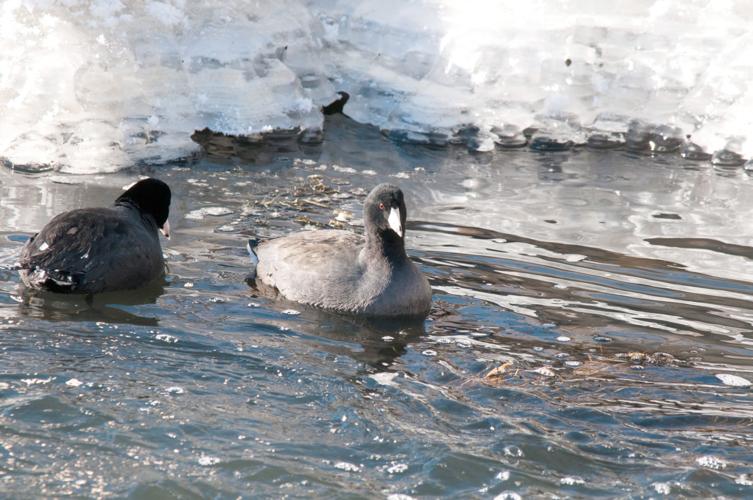The image depicts a vibrant outdoor scene with a focus on natural elements, primarily water. The water appears slightly choppy, featuring numerous waves and ripples that reflect the sunlight. The surface shows hints of sea foam, and the color is predominantly a grayish blue, adding to the dynamic texture of the scene. Towards the far end of the image, the water meets a stretch of ice, which is illuminated by sunlight, casting both light and shadows across its white expanse. In the foreground, the image centers on two ducks. One duck, positioned centrally and slightly toward the right, faces the camera in almost a side profile. This duck showcases mostly light gray feathers with a darker gray head and sports a white beak and a visible brownish-orange eye. To the left, a second duck faces away from the camera, revealing more of its darker gray body and a blackish head, along with a partial view of a white beak. The sky is clear, emphasizing the sunny conditions that create various reflections on both the water and the ice.